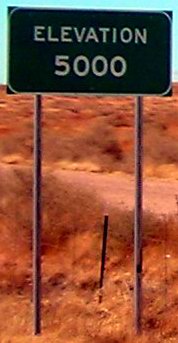This photograph captures a high desert scene featuring a street sign that reads "Elevation 5,000" in white font on a dark green rectangular background with a white border that has curved edges. The sign is mounted on two tall metal poles. Above the sign, the sky is a striking turquoise, while below and in the background, the landscape is dominated by earth tones with shades of gray, orange, red, and yellow. There are scattered dead bushes, brush, and shrubs, with a red sandy path and hints of a wire fence visible in the distance. The overall scene conveys a dry, desert environment featuring rocky terrain and sparse vegetation.